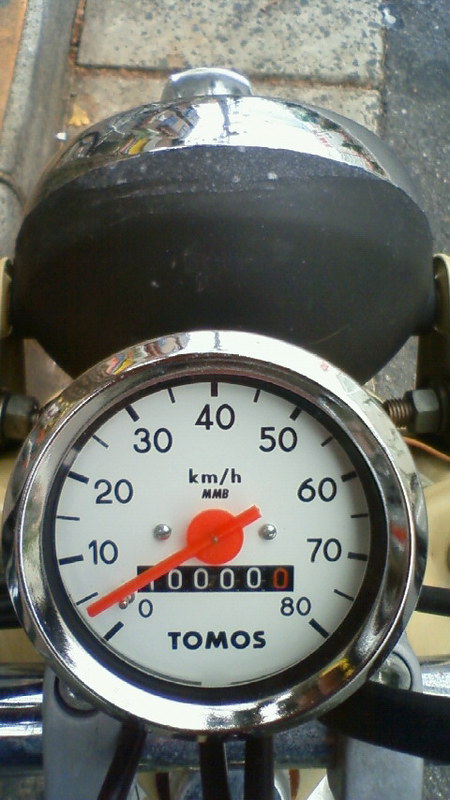This close-up photograph captures a highly detailed view of a speedometer mounted on a recreational vehicle, likely a motorbike. The circular speedometer features a sleek silver outer casing and a white inner face adorned with black numbers, indicative of the current speed in kilometers per hour (KM/H). Prominently displayed in the center, the "MMB" logo signifies the make of the speedometer. The numbers, starting from 0 and ascending in increments up to 80, are accompanied by precise slash marks for more detailed readings. The orange needle points to the current speed, while a small mileage tracker beneath the needle records the total miles driven. Just below this tracker, the brand name "Tomos" clearly identifies the manufacturer of the vehicle. The device is securely fastened by two screws positioned symmetrically beside the needle.